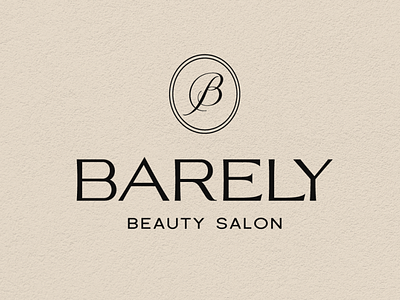The image is a logo, likely for a business, set against a light beige background with no borders. Dominating the center is an elegant, script letter "B" in black. Surrounding the "B" is a black oval composed of two concentric lines, adding a touch of sophistication. Beneath this emblem, the word "BARELY" is displayed prominently in large, black, capital letters. Below "BARELY," the words "Beauty Salon" are shown in smaller, black letters. The design is elegantly simple and clearly identifies the business as the Barely Beauty Salon.